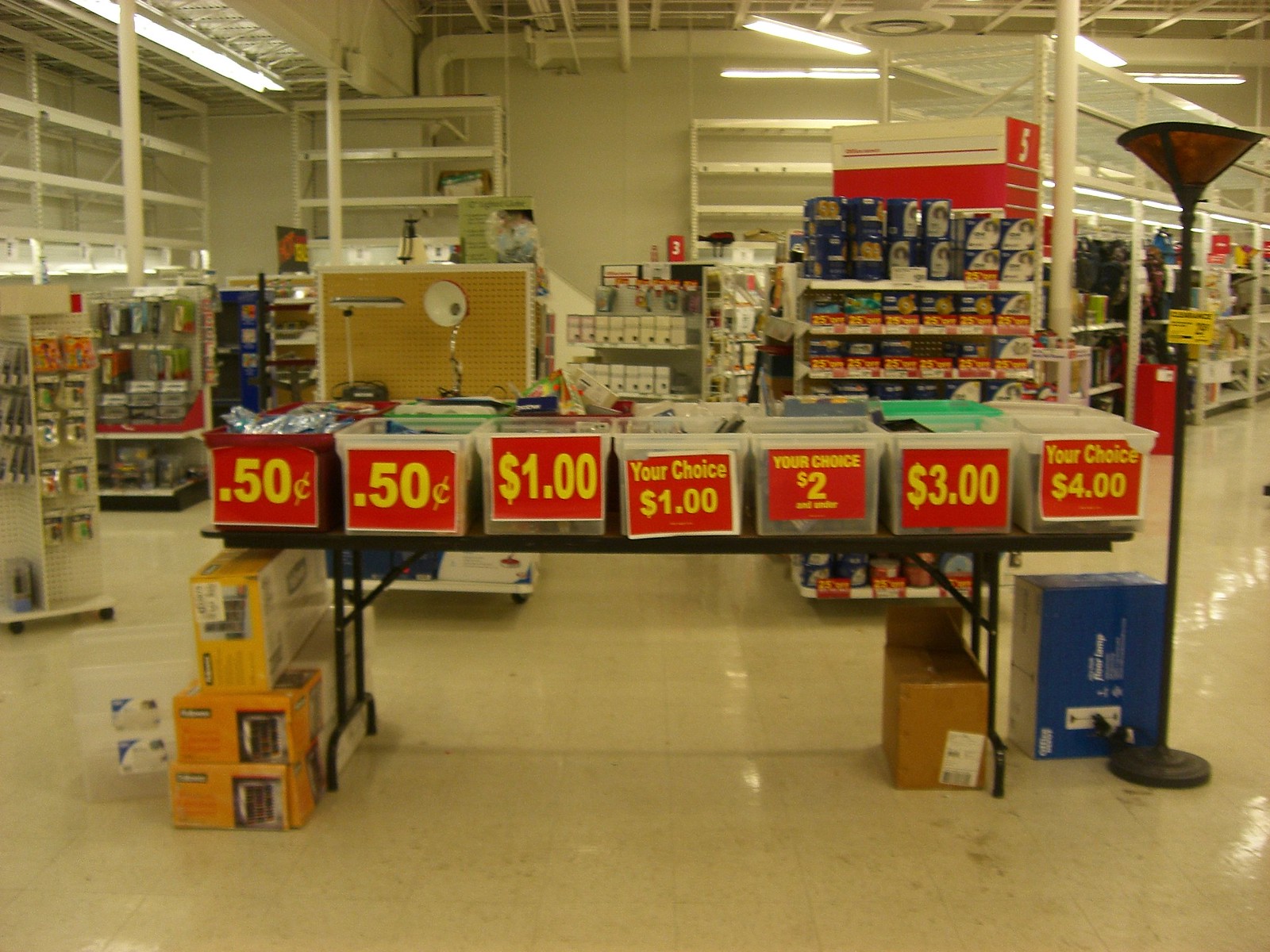The photograph captures the interior of a retail store, characterized by its plain white back wall and warehouse-style ceiling, with long fluorescent lights hanging down. In the foreground, prominently featured, is a folding table with metal legs, topped with clear plastic storage bins labeled with various prices: $0.50, $0.50, $1, your choice $1, your choice $2, $3, and your choice $4. These large red signs with yellow writing indicate the bins' bargain prices. To the right of the table stands a tall floor lamp with an upward-facing, cone-shaped brown shade and a tag attached. The scene extends beyond the table where orderly rows of shelves display a variety of small items, cans, blue canisters, and boxes, detailedly organized to the left and right of the table. Various stands hold hanging items, with some sections appearing empty, while blue and yellow boxes and additional product shelves create a bustling retail environment.